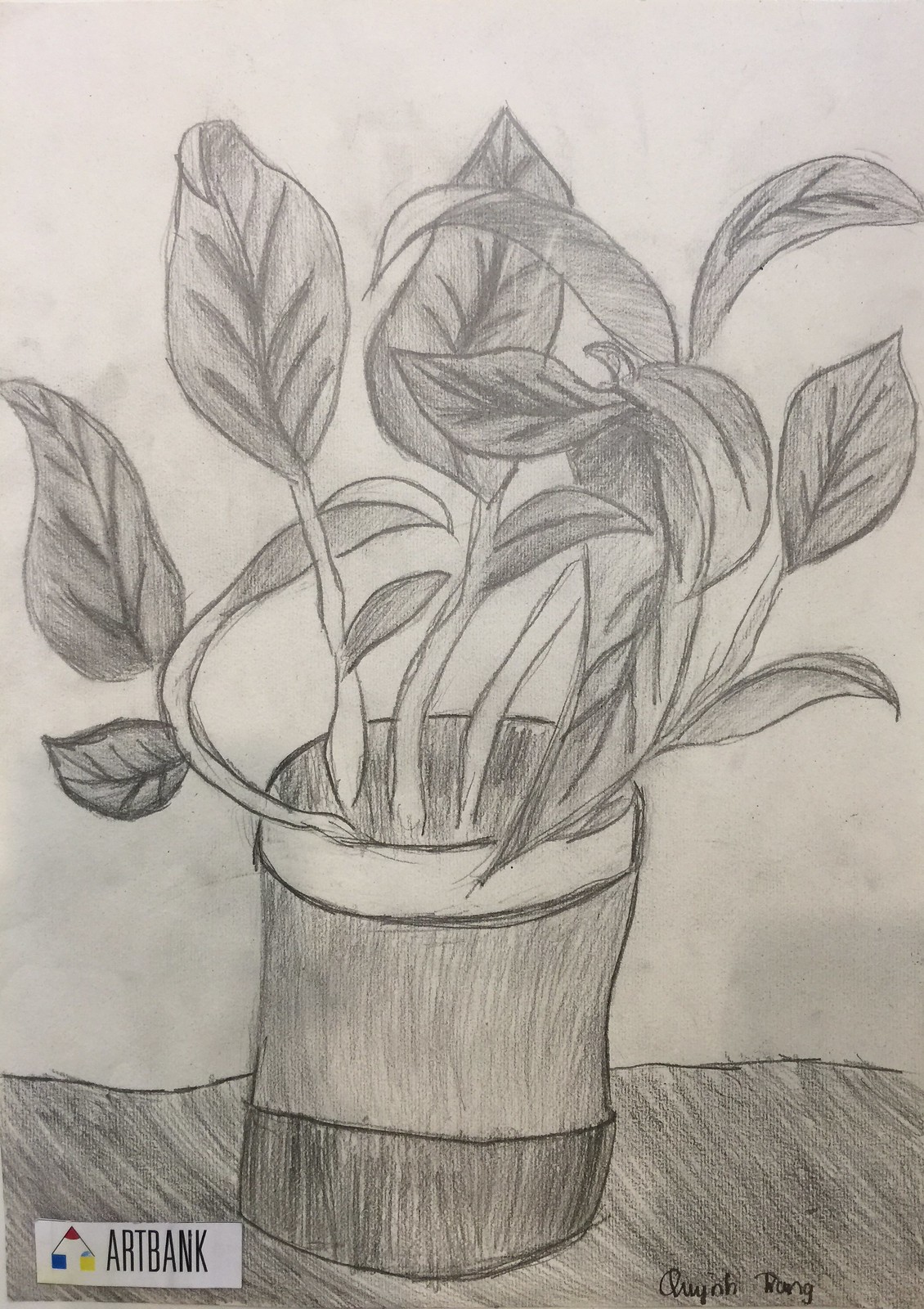A detailed heavy pencil drawing dominates the entire photograph, showcasing an intricate depiction of a plant in a planter. The planter is cylindrical and rests on a shaded, irregular table surface, adding depth and texture to the composition. The stems emerge from the planter, culminating in large, oval-shaped leaves with pointed tips. These leaves exhibit a dynamic quality, curling and wrapping around each other in various sizes, adding a sense of movement to the piece. The background features smudged gray shading, enhancing the prominence of the plant and creating a subtle contrast. In the lower right corner, the drawing is marked with the phrase "Art Bank" accompanied by a logo. The artist's signature is also present at the bottom right, completing the composition with a personal touch.